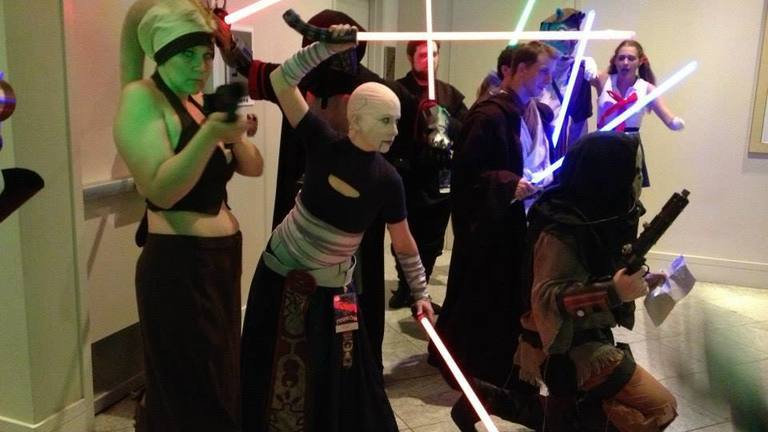This detailed horizontal photograph captures an indoor scene likely set in a large room with white walls and a tiled floor, possibly a retail building due to a visible door with a silver push button. The image depicts a Star Wars-themed costume party with various individuals dressed in elaborate costumes, wielding glowing lightsabers.

Centrally positioned is a striking figure appearing in a black short sleeve fitted top featuring a cutout above the breast. She dons a bald cap and facial makeup, including white paint which matches her striped, bandaged belt and brown skirt. Her dynamic pose showcases her holding two lightsabers - one in each hand - with her right arm raised above her head and her left arm bent and extended sideways.

In the foreground, there's a person kneeling on the ground, dressed in a brown ensemble with a black hood that covers their head and neck, obscuring their face. This individual holds a revolver in their right hand and something else in their left hand. Their profile, along with the woman’s, is directed towards the right side of the picture.

Additional figures populate the background, including a woman wearing a black headband, black tank top, and a skirt or pants, seemingly taking a photograph. Another notable presence is a woman on the left, clad in a vest crop top, low-waist skirt, and a large head covering resembling a sock, also holding a gun.

The scene is lively and detailed, with several individuals holding lightsabers resembling those from a science fiction movie. The combination of costumes and props effectively conveys a distinct Star Wars ambiance, enhancing the festive and themed atmosphere of the gathering.